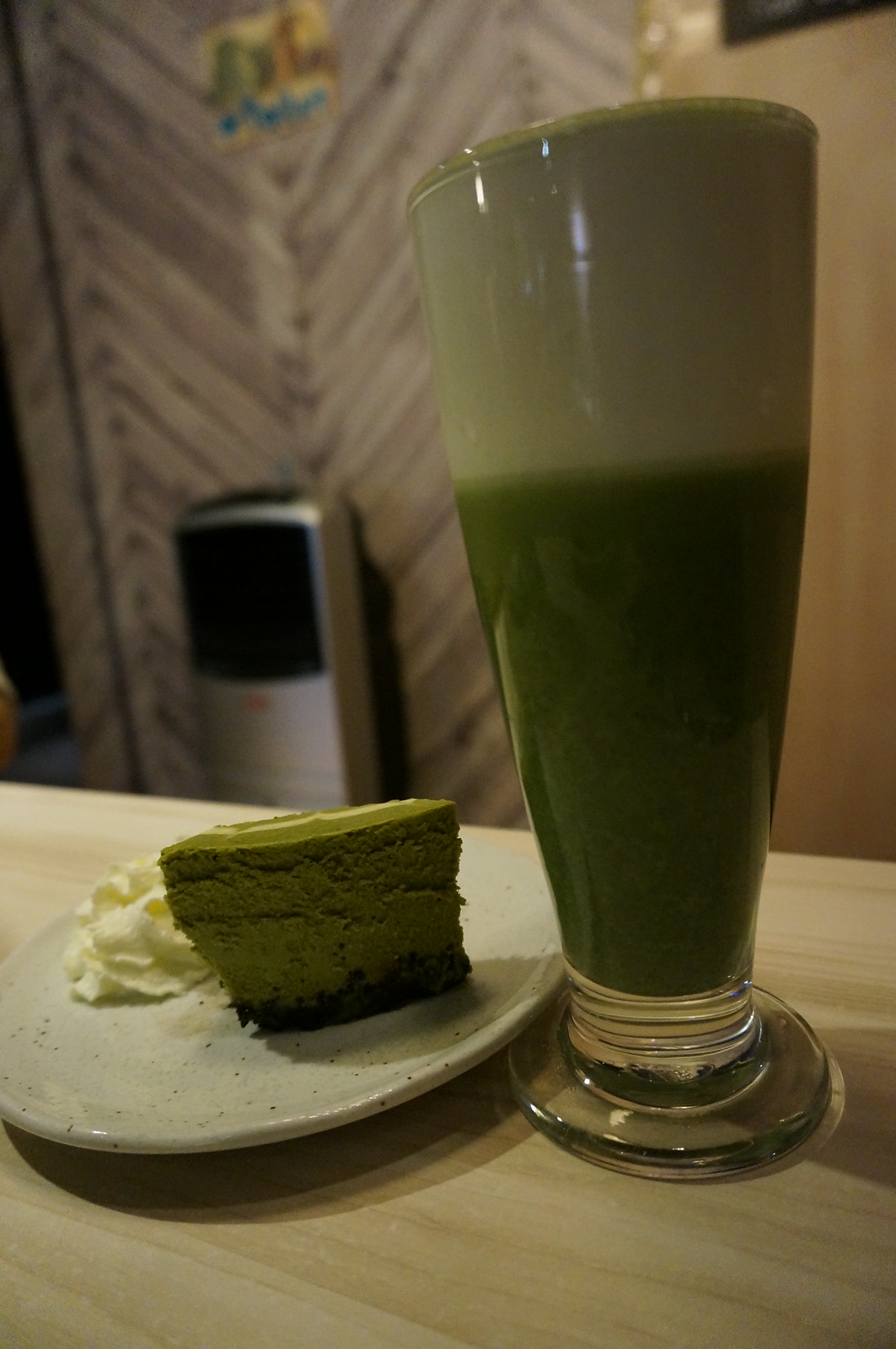In the photograph, we see a vibrant lime-themed arrangement displayed on a light wooden table. To the right, there is a tall, narrow Pilsner-style glass containing a lime drink. The beverage fills up about three-quarters of the glass, topped with a layer of white foam. The drink's color suggests a refreshing and possibly lime-flavored concoction. Adjacent to the glass, on a white speckled plate, sits a delicious lime pie with a chocolate crust. The pie is garnished with a dollop of vanilla whipped cream and a small decorative flower made of frosting. The scene is softly lit, with subtle reflections playing off the glass surface. The background, though out of focus, reveals some type of freestanding device against the wall, adding a touch of environmental context. This detailed setup evokes a sense of a festive or themed tradition, perhaps even reminiscent of St. Patrick's Day with its green hues and celebratory arrangement.